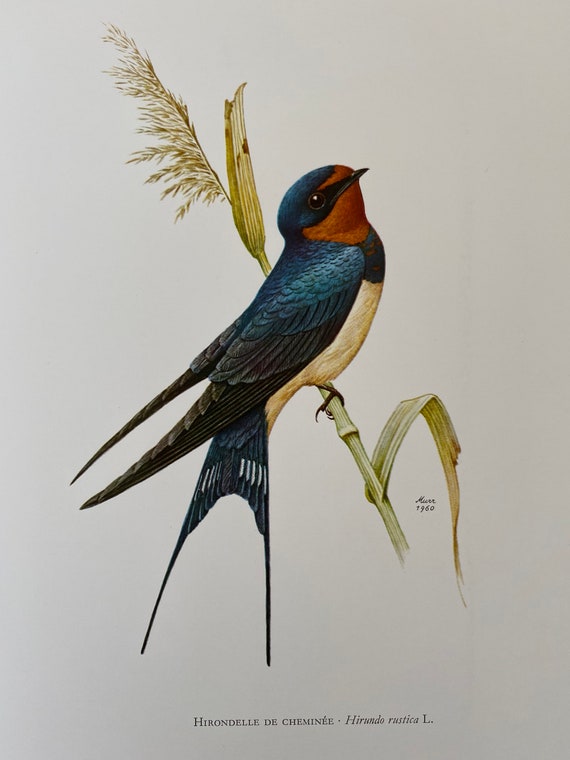This detailed artist's illustration features a stunning bird perched centrally on a piece of wheat or straw against a plain white background. The bird, identified by the text below the image as "Hirondele de Chimene," exhibits a rich coloration: blue feathers that fade into darker blue and black along its wings, a brown face with a small black beak, and a white underbelly. Additional text beneath the bird, rendered in small, difficult-to-read script, includes a date, 1958. The bird is magnificently detailed, with intricate feather patterns and lifelike posture, providing a vivid and captivating depiction of this exotic species. The wheaten perch adds a natural element, enhancing the overall aesthetic of this elegant illustration.